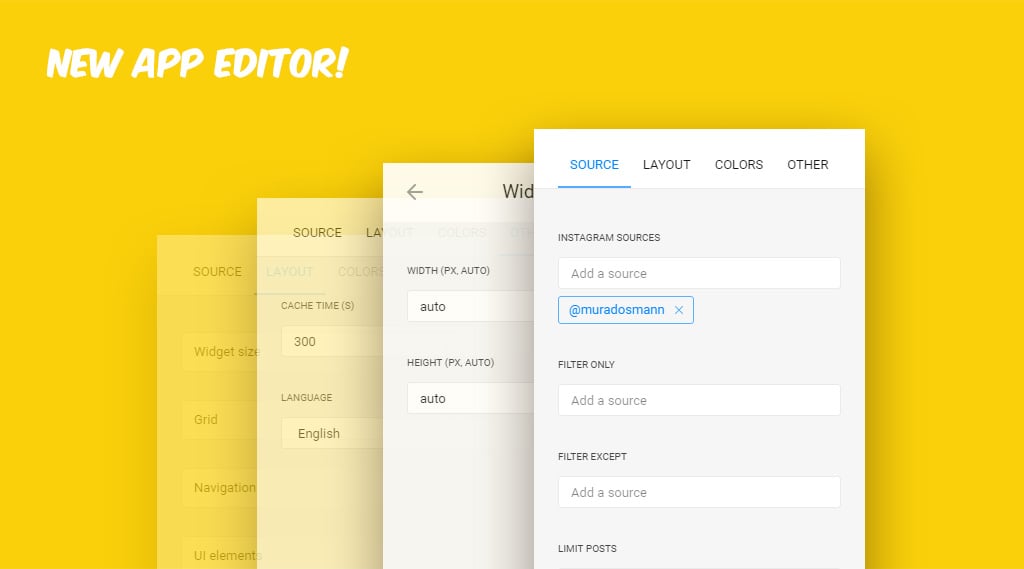### Detailed Caption:

The image appears to be an advertisement for a new mobile application editor. It features a striking yellow background that is pure and unblemished, providing a vibrant and eye-catching canvas. At the top left corner in bold, white, all-capital letters, the text announces "NEW APP EDITOR!" with an exclamation mark for emphasis.

Central to the graphic is a series of four mobile device screenshots presented in an overlapping manner. The leftmost screenshot is rendered smallest and most transparent, creating a visual gradient towards the fullest and most opaque image on the far right. This progression symbolizes depth and focus, drawing the viewer's attention to the detailed functionalities of the app.

On the fully visible rightmost screenshot, a menu at the top showcases four navigation tabs labeled "Source," "Layout," "Colors," and "Other." Underneath this menu, the interface displays options for managing Instagram sources. There is a designated field for entering a username, shown in the example as "Murad Dosman." Additional functionalities include "Filter Only" and "Filter Except," each with corresponding input fields for other usernames. Finally, a "Limit Posts" option provides further customization, reinforcing the editor's robust capability to tailor social media content effortlessly.